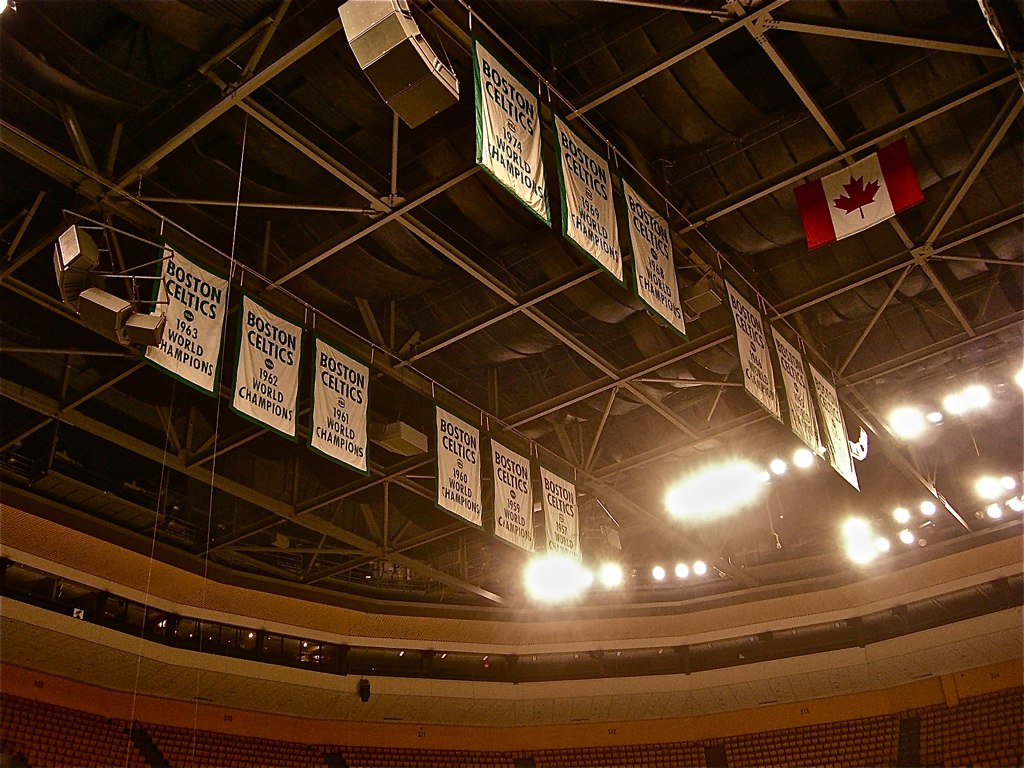The image captures the interior ceiling of an indoor sporting stadium, identified as the home arena of the Boston Celtics. Suspended from the exposed metal and steel rafters are 12 white championship banners arranged in two rows of six. Each banner proudly displays "Boston Celtics," followed by a year commemorating their championship titles, and the phrase "World Champions" below that. The years of victory visible in the image include 1951, 1958, 1959, 1961, 1962, 1963 in the back row, and 1974 and 1979 in the front row, though some banners in the foreground are partially obscured. Adding to the visual narrative is a Canadian flag with its distinctive red maple leaf, hanging separately on another rafter. The stadium's upper levels, including skyboxes, brown-shaded upper bleachers, and third-level seats, are discernible in the background. Bright spotlights attached to the ceiling illuminate the structure, enhancing the view of the intricate beam work supporting the roof.